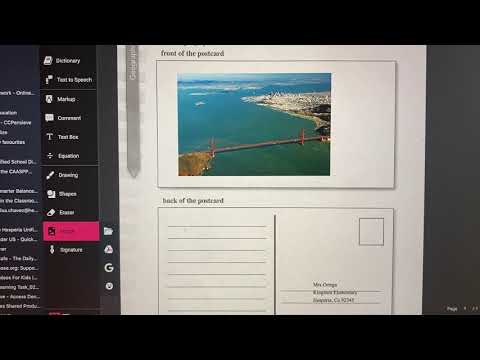Displayed on the computer screen is the image of a postcard. The postcard prominently features a scenic view of a large bridge spanning over a body of water with what appears to be a distant cityscape, suggesting a city on the water. The bridge is notably smaller in the frame, possibly taken from a high vantage point like a helicopter. The overall backdrop of the postcard image includes a wide expanse of blue ocean, flanked by ground on either side of the bridge.

Below the main postcard image, there are lines designated for writing messages and sections for the name and address. The text on the postcard is quite small and mentions the "front of the postcard" and "back of the postcard."

To the left of the postcard image, the computer screen displays several menu options in white text on a black background, including "dictionary," "text to speech," "markers," "comment," "text size," "equalizer," "drawing," "shapes," "eraser," and "signature." A pink bar highlights one of these options, although it isn't fully legible. The overall scene depicts a digital interface for creating and customizing postcards, combining both graphic elements and functional tools for user interaction.